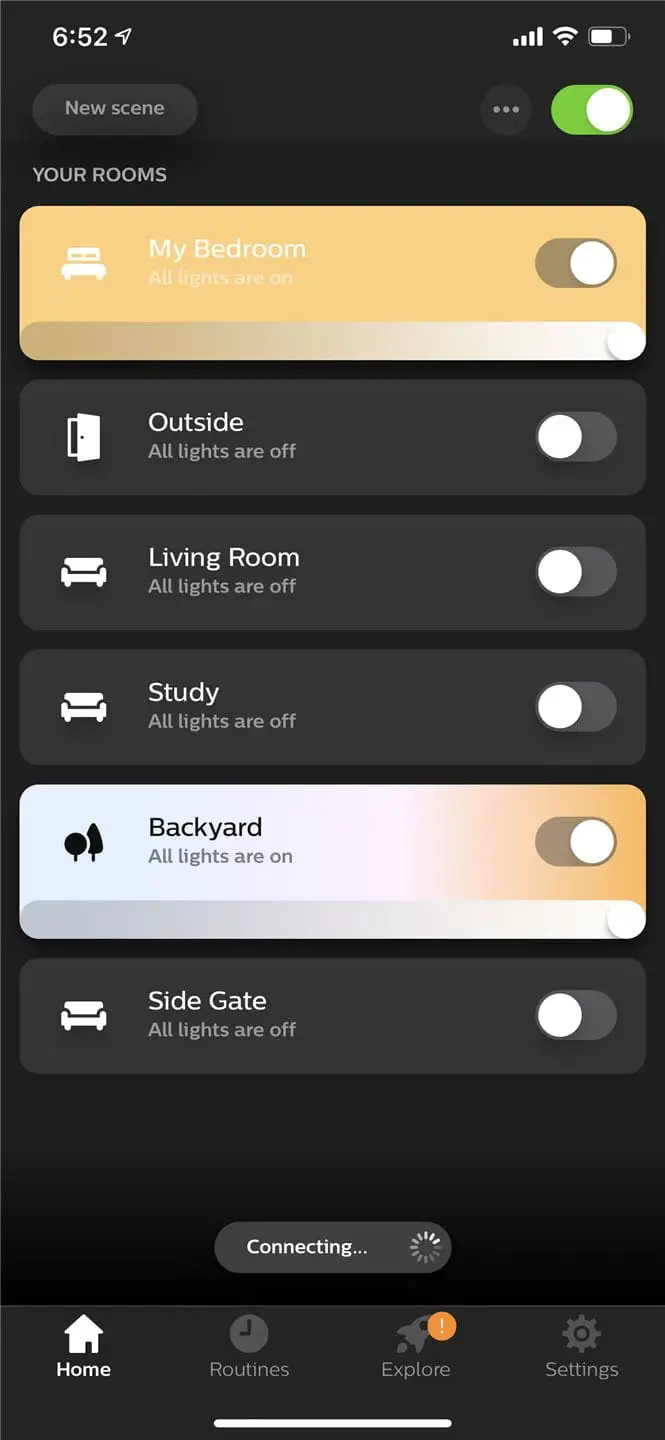In the detailed image of a cell phone screen, we observe the following elements:

1. **Battery and Connection**: The battery icon shows approximately 75% charge. To the left of the battery, “652” indicates the connection strength.

2. **Current Scene**: The screen displays the "new scene" in lighter gray text.

3. **Toggle Switches and Headings**: 
   - **Your Rooms**: This category is displayed with an active green switch, turned to the right.
   - **Bedroom**: Highlighted in orange with an icon of a bed, indicating "All lights are on".
   - **Outside**: All lights are off as shown by accompanying icons.
   - **Living Room** and **Study**: Both show all lights off, highlighted by their respective icons.

4. **Detailed Descriptions for Each Room**:
   - **Backyard**: Highlighted and states "All lights are on" with an illustration of two trees.
   - **Side Gate**: Indicates "All lights are off" with an image of a gate.

5. **Connection Status**: At the center, there is the word "Connecting" with a spinning cursor indicating the device is attempting to connect.

6. **Navigation Bar at the Bottom**:
   - **Home**
   - **Routines**
   - **Explore**: Noted with an orange circle containing the number 1.
   - **Settings**
   - The bottom portion has a white bar.

This detailed description captures the interface's layout and the status of various elements within the smart home control application on the cell phone.